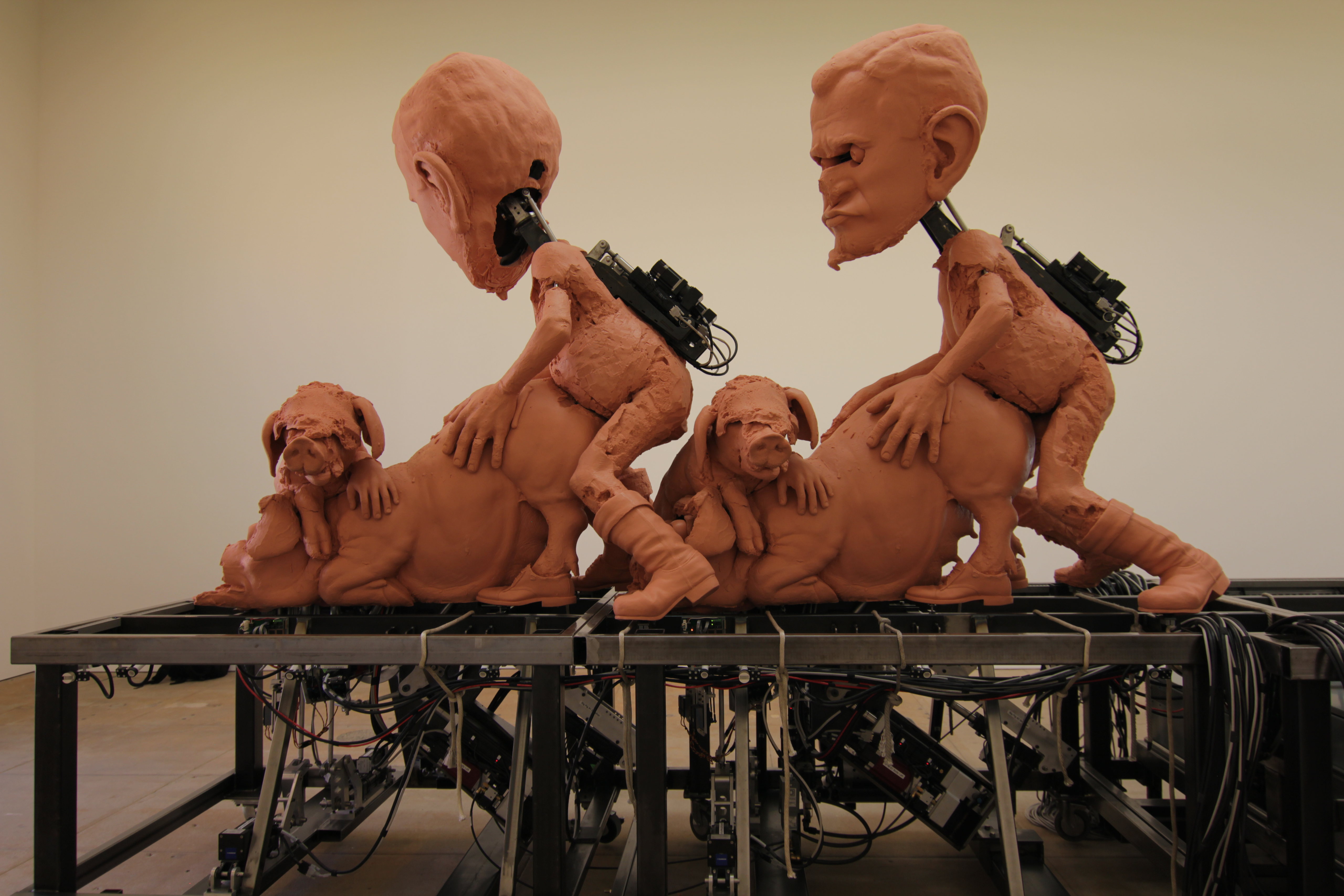This is a highly detailed color photograph showcasing a provocative animatronic art installation set against a plain white backdrop. The scene is centered on a metal platform crowded with visible gears and wires, lending an industrial feel to the artwork. The startling focal point features a female sow pig positioned with her face down and front paws bent, her rear conspicuously arched upward. Draped over her neck lies a baby piglet, adding a layer of vulnerability to the scene. 

Behind her, a menacingly expressive male figure is grasping her hips, reenacting an aggressive stance suggestive of forced sexual activity. This unsettling tableau is mirrored directly behind them with another male animatronic figure, similarly clutching the sow's hindquarters in a forceful manner, his face twisted into a threatening expression. Notably, the pigs in this installation are sculpted in a pink hue reminiscent of clay, and one noticeable detail is the shoes adorning the hind feet of the piglets.

Additional complexity is added by metallic packs strapped to the backs of the male figures, bristling with wires that evoke an impression of explosive devices, thereby heightening the tension and sense of violation in the artwork. The entire arrangement may serve as a poignant commentary on humanity's exploitation and mistreatment of animals for selfish purposes, wrapped in an unsettling portrayal of violent subjugation.